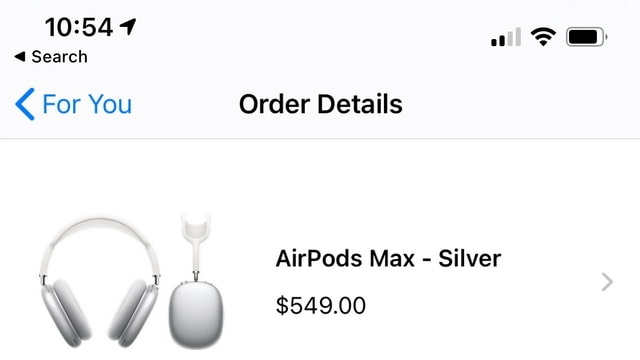Screenshot of a smartphone displaying a webpage detailing an order for AirPods Max in Silver. 

At the very top, the smartphone interface shows the time as 10:54 with an upward-pointing arrow, possibly indicating airplane mode. The connectivity status displays two out of four bars, alongside a Wi-Fi symbol, and a battery level at approximately 90%.

Just below, a blue left-facing arrow and blue text reading "For You" signify a clickable link. Centralized beneath this, "Order Details" is prominently displayed, followed by a thin divider line.

The main content features images of AirPods Max, depicting two angles: a full frontal view showcasing both ear cups and the looped headband, and a back view of one ear cup, offering a different perspective.

Adjacent to these images, the text "AirPods Max - Silver" is displayed along with the price, $549. To the right, a gray right-facing arrow indicates further interaction or navigation options.